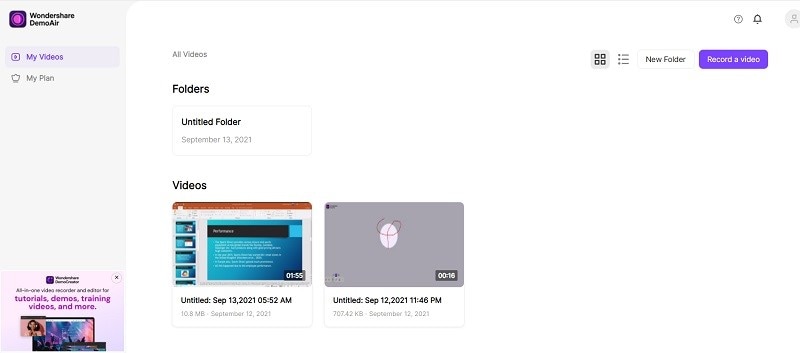The image displays the interface of the Wondershare Demo app, identifiable by its prominent purple and pink circle symbol. At the top of the interface, the app name "Wondershare Demo" is displayed, followed by several tab labels. The bottom menu includes options such as "My Videos," "My Plan," "All Videos," "Folders," and "Untitled Folder - September 13th, 2021." Below these options, there are sections labeled "Videos," showcasing two video files.

The first video, created on September 13th, 2021 at 5:02 a.m., is unnamed and has a file size of 10.8 megabytes, with a duration of 1 minute and 55 seconds. The second video, also unnamed, was created on September 12th, 2021 at 11:46 p.m., has a shorter duration of 16 seconds, and a file size of 707.42 megabytes.

The interface allows for different viewing formats: a square grid view or a list (bullet form) view, which can be adjusted using controls located to the top right of the video list. On the far right, there are options to create a new folder and a purple button labeled "Record."

Adjacent to these controls, at the top right corner, are icons for additional app functionalities, including a question mark for help, a notification bell for alerts, and a profile picture, indicating user account options.